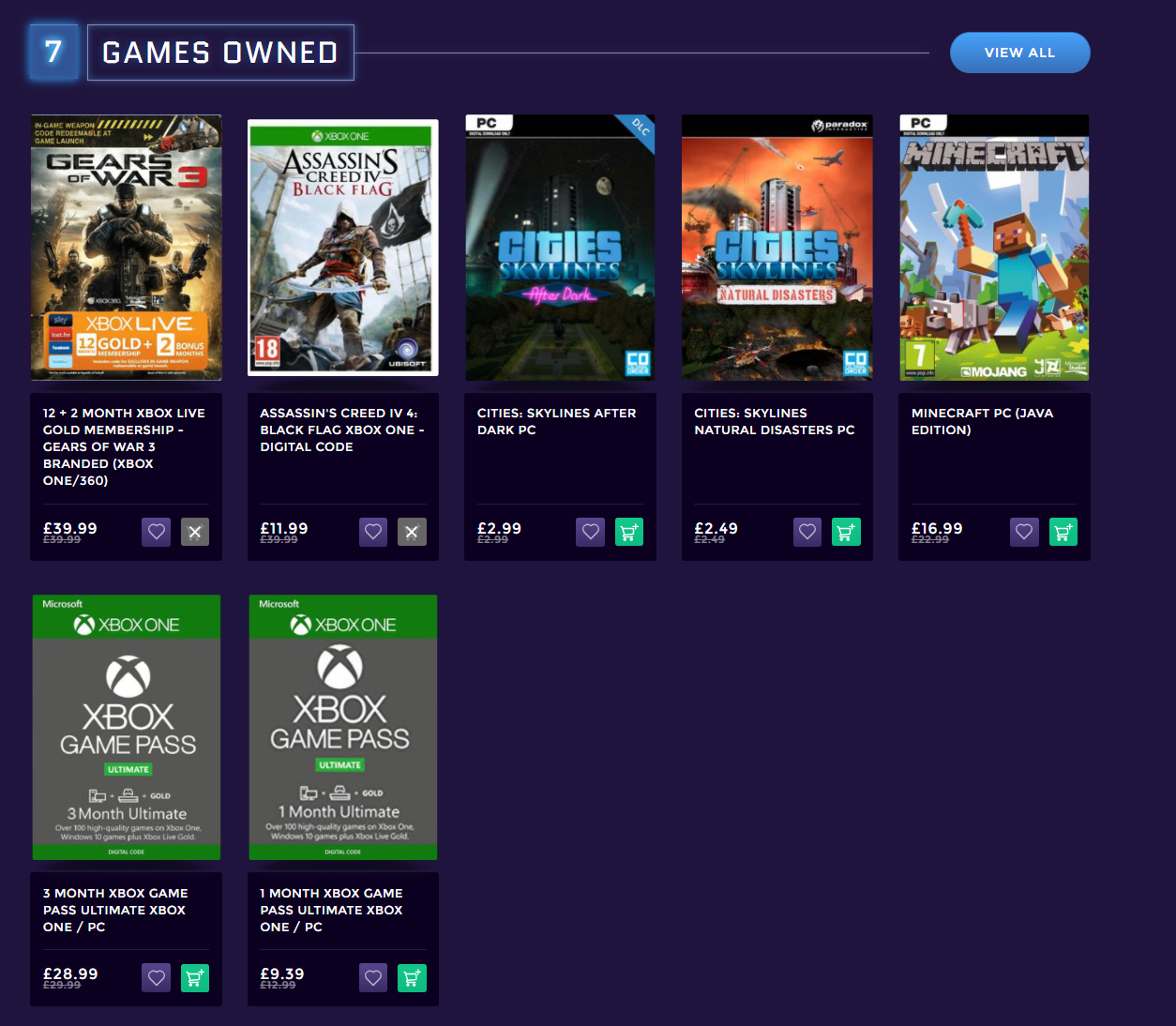The screenshot showcases a game library interface set against a black background. In the upper left corner, a blue box prominently displays the number seven, indicating the total number of games owned. Adjacent to it, a labeled rectangle reads "Games Owned," while a blue "View All" button is situated on the far right.

The main section of the interface features two rows of displayed game covers. The first row consists of five game covers: 

1. "Gears of War 3" is positioned in the upper left, depicting a soldier with a dramatic sky backdrop and marked with "Xbox Live Gold" at the bottom front.
2. Next to it is "Assassin's Creed IV: Black Flag," featuring a soldier with a black flag billowing behind them.
3. To its right, "Cities: Skylines" is shown, presenting a night view of a cityscape.
4. Continuing right, another "Cities: Skylines" game cover appears, this time showcasing an orange sky with a prominent gray building.
5. The last game in the row is "Minecraft," characterized by its iconic pixelated art style and a character with a black head, blue shirt, and pickaxe, set against a blue sky backdrop.

The second row contains two items labeled "Xbox Game Pass." Both covers feature a green top section and a gray background with "Xbox Game Pass" written on the gray portion. 

The layout and vivid imagery give a comprehensive overview of the user's game library.